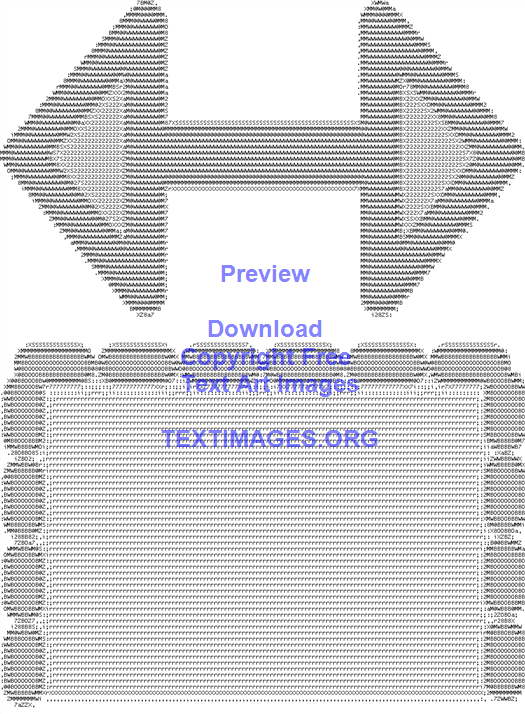The image showcases a predominantly gray color scheme and features two distinct sections. The upper part consists of an arrow-like structure pointing in both left and right directions simultaneously, with two solid triangles on either end of a connecting line, resembling the shape of a dumbbell. Below this arrow formation, blue text displays the words "preview, download, copyright free, text, art, images, and textimages.org." Underneath this text, there is a rectangular shape with several smaller, tube-shaped or tic-tac-like darker forms along the top, left, and right edges, leaving the bottom devoid of any such shapes. The overall design appears simple and pixelated.